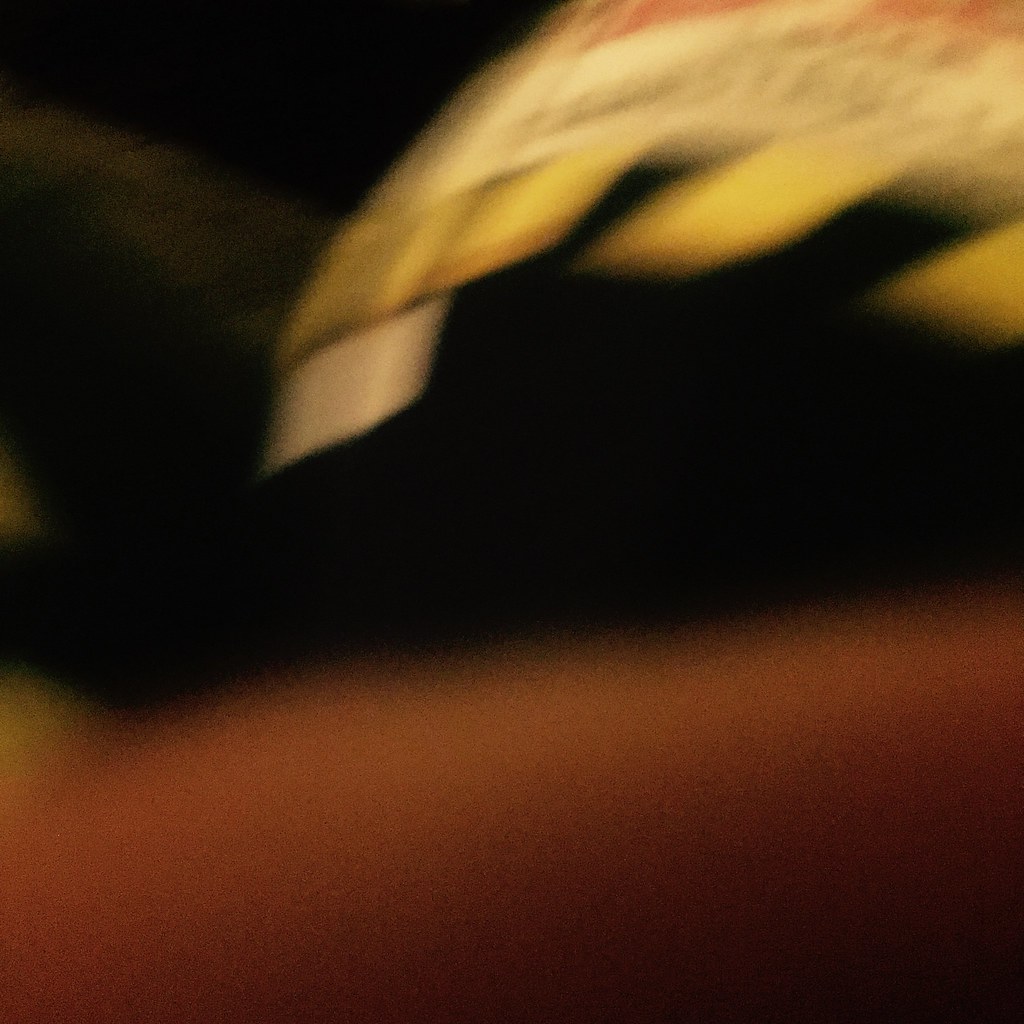In this semi-dark, blurry photograph, the main focus lies in the upper right-hand corner, where an object with yellow teeth-shaped grips or gears can be seen. This object bears some writing and is attached to a white and red curved structure, which culminates in a larger white tooth-like feature at its tip. In the bottom portion of the image, there's a very blurry and shaded human Caucasian forearm, creating an impression of depth and subtle movement. The background showcases dark areas that further accentuate the semi-dark setting. On the left-hand side of the photo, shades of darker yellow and green blend into the scene, contributing to the overall color palette. Near the crook of the person's elbow, there appears to be the faintest hint of a yellow t-shirt.